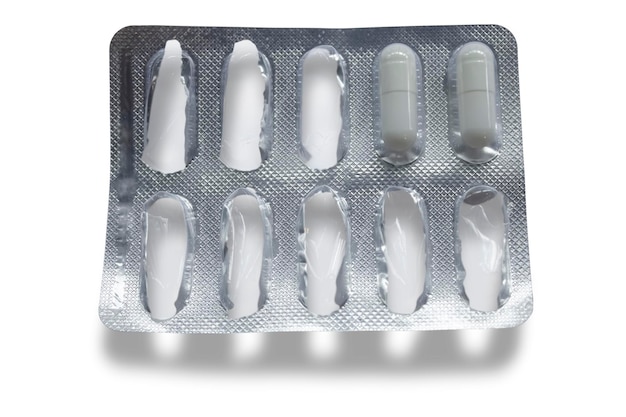This image features a rectangular, silver foil pill pack with ten individual pouches, set against a solid white background with a shadow suggesting overhead lighting. Eight of the pouches have been used, leaving only two white pills remaining. The package contains three empty pouches on the top row and five fully used pouches on the bottom row. The two remaining pills, encased in clear plastic domes, are white with a divider down the middle, suggesting they may contain a white powder. The foil packaging is devoid of any labels, names, or logos, making it indistinguishable as either a prescription or over-the-counter medication. The packaging appears standard, with rounded corners and no identifying marks.